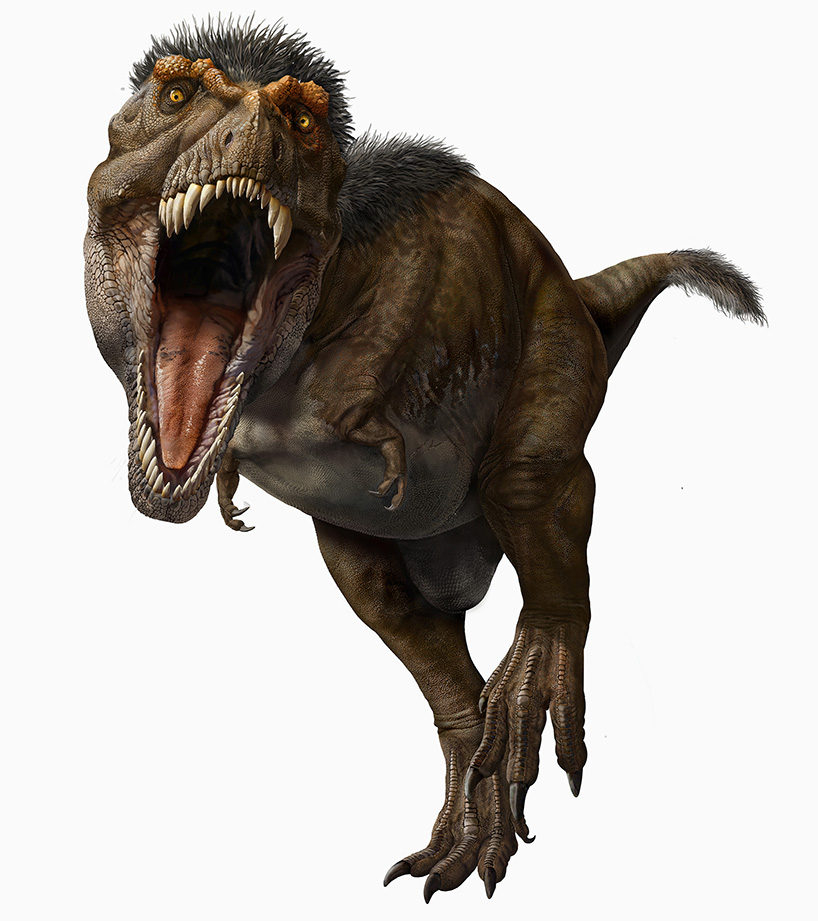The image depicts a dinosaur, resembling a T-Rex, set against a very light gray or white square background. The dinosaur's head is positioned in the upper left corner of the frame, and its body extends diagonally towards the bottom right, where its feet and tail end. The dinosaur's face is prominently large, directly facing the viewer with an open mouth full of razor-sharp, pointy teeth in both the upper and lower jaws, and an elongated, pink tongue with black specks inside. 

The creature's eyes are a striking gold or yellow, and it has medium brown or Dijon mustard-colored eyebrow ridges. The top of its head and upper back are adorned with little spikes of black or dark brown fur that continue along its back and onto its tail, which is relatively short and also furry. The dinosaur's overall body coloration is a dark, muddy brown with black stripes and spots, and its underbelly is a contrasting white or gray.

Its stance is dynamic, as if running towards the front of the image, with its left leg raised and bent, and its right leg firmly placed down, showcasing large feet with three formidable claws each. The arms are notably tiny, barely extending from under its belly, each ending in small claws. This combination of features makes the dinosaur appear both ferocious and ready to leap out of the frame.